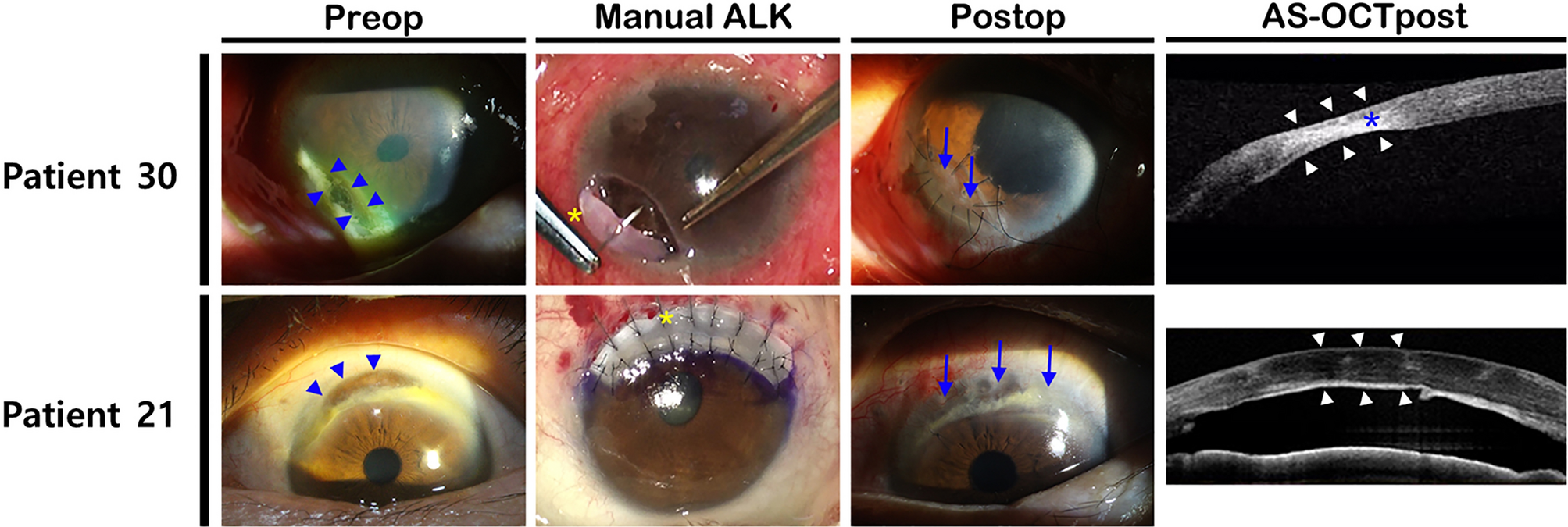This image displays a series of eight color-coded and labeled ophthalmic photographs arranged in a 2x4 grid. The top row is labeled "Patient 30," and the bottom row is labeled "Patient 21." Above each column, the headers read, from left to right: "Pre-op," "Manual ALK," "Post-op," and "ASOCT Post." The first six images show detailed eye pictures, with the pre-op images featuring blue triangles highlighting specific areas. The manual ALK images depict surgical tools and techniques, implying ongoing surgical procedures, while the post-op images illustrate the results with blue arrows pointing out key changes. The final column consists of black-and-white, x-ray-like images displaying nerve structures, marked with white arrows.